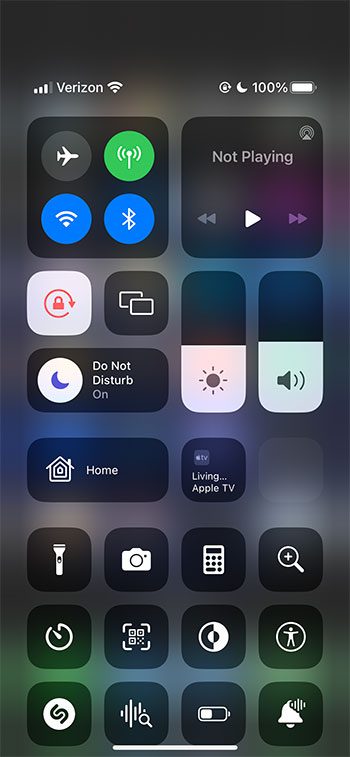The image displays the settings overlay pulled down from the top of a cell phone screen, superimposed on the home screen's wallpaper. The background is predominantly dark, transitioning to black at the top, with hints of green, purple, blue, and white hues—likely the icons from the home screen showing through the semi-transparent overlay.

In the top-left corner, the status bar indicates "Verizon" with three or four signal bars and a full Wi-Fi indicator. On the upper right, there is a crescent moon icon next to a 100% battery indicator.

The overlay contains various black boxes housing different icons. The first box in the upper left features icons for airplane mode, a broadcast signal, and Wi-Fi and Bluetooth connections represented by green and blue bubbles, respectively.

A section labeled "Now Not Playing" appears, accompanied by play, skip, and backward buttons. Below, additional icons include a lock icon, a "Do Not Disturb" toggle, and adjustable options for brightness and sound. There are also buttons labeled "Home" and "Living Apple TV," along with icons for a flashlight, camera, calculator, plus sign in a magnifying glass (probably a search function), and others suggesting accessibility options, contrast settings, and audio controls. Additionally, there is another battery indicator and a notification settings icon.